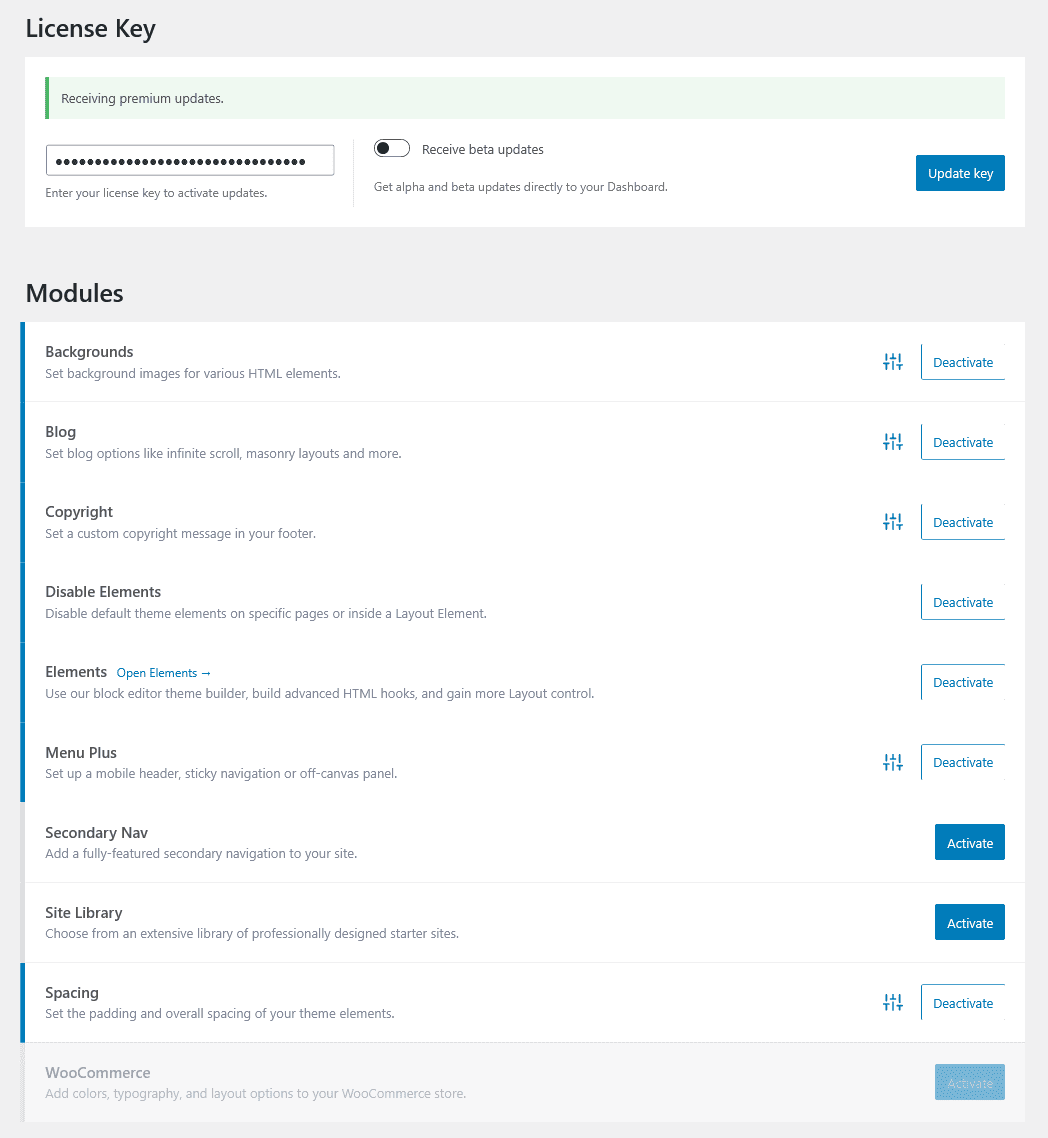This screenshot captures a detailed view of a licensing and features management webpage for a software product. At the top left corner, the text "License Key" is prominently displayed, signifying the section's purpose. Directly beneath this, a green notification banner reads "Receiving premium updates," indicating that premium updates are in effect. Below the notification is a text box, partially filled with obscured characters (dots), where a user has entered their license key.

Next to this text box is an option labeled "Receive beta updates," which remains unselected, as indicated by its default color not changing to signify activation. To the far right of this section, there's an "Update Key" button.

Below the license key section, there is a list of modules featuring the following entries: Backgrounds, Blog, Copyright, Disable Elements, Elements, Menu Plus, Secondary Nav, Site Library, Spacing, and WooCommerce. Except for "Secondary Nav" and "Site Library," all modules display a "Deactivate" button on the right, indicating they are currently active. The "Secondary Nav" and "Site Library" modules show an "Activate" button, suggesting they are not activated at this moment.